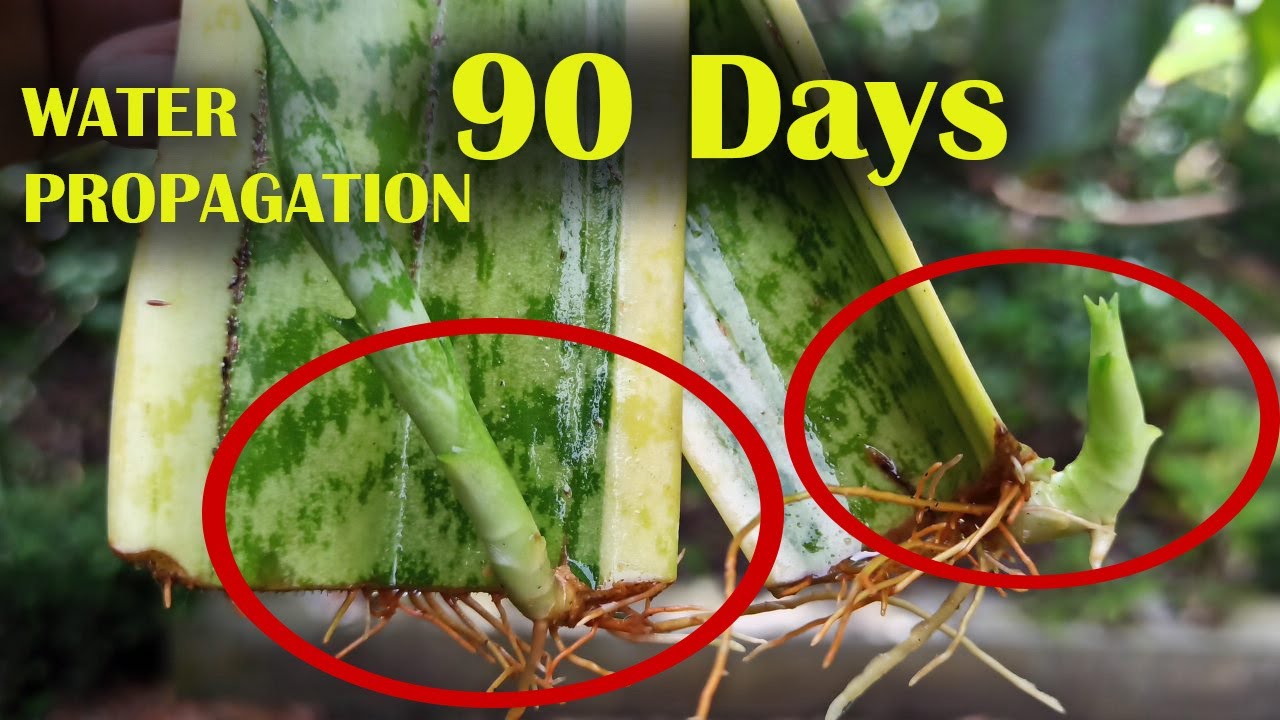The image showcases two aloe vera plants that have been propagated in water for 90 days, emphasizing the significant root development achieved in this period. The picture features bold yellow text that reads "Water Propagation 90 Days," with a thick, light and opacity drop shadow for added emphasis. The image is sharply focused on the plants and their extensive, healthy, pale-colored roots, which are circled in red for clarity. The roots are slightly slimy, suggesting a need for a water change. The background is a blurred blend of green foliage and a concrete slab, providing a lush, out-of-focus contrast to the detailed foreground.